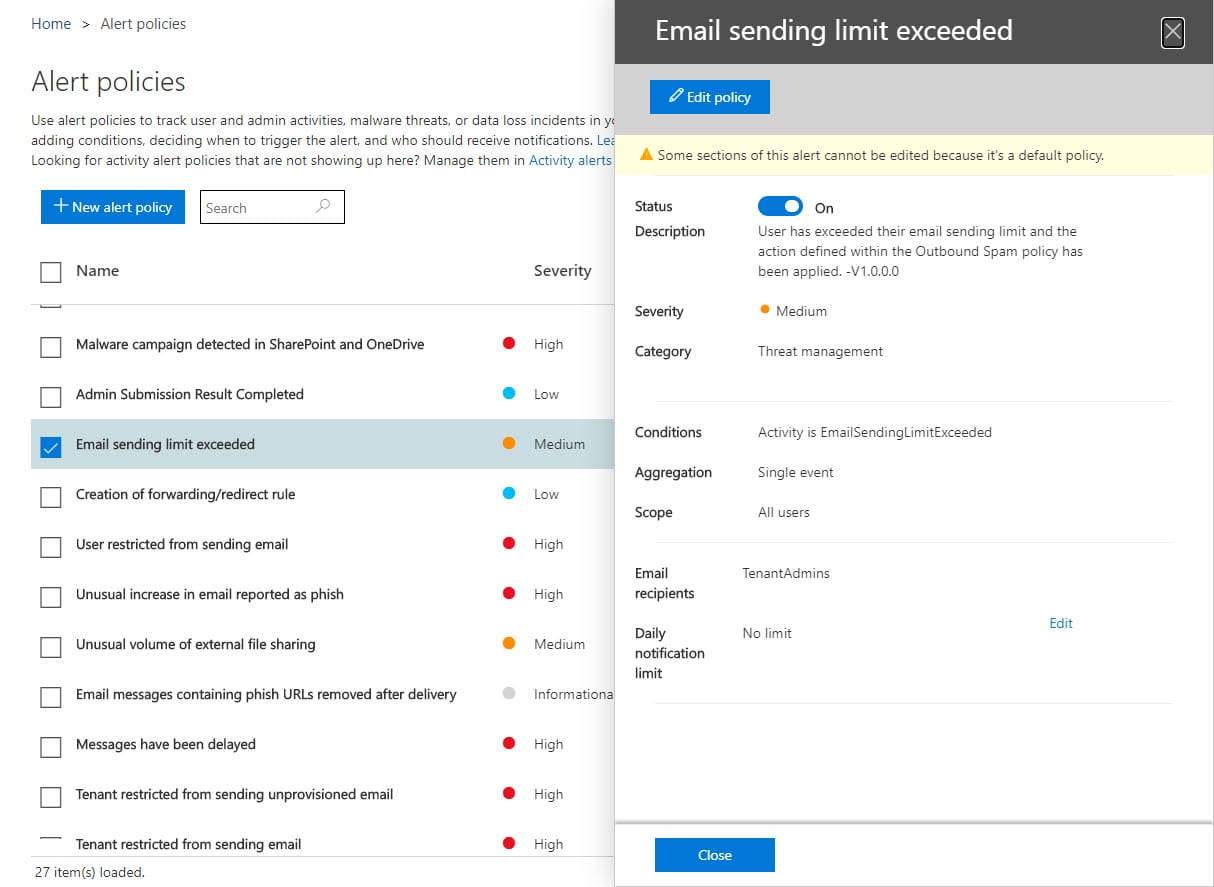**Websites** 

The section features two side-by-side images of an alert management system.

1. **Left Image: Alert Policies Overview**
   The left image displays a section titled "Alert Policies" with instructions on using alert policies to monitor user and admin activities, tackle malware threats, or manage data incidents. The guidance explains the process: add conditions, determine trigger criteria, and specify who receives notifications. Users are encouraged to manage their activity alerts in the "Activity Alerts" section. A prominent blue button labeled "New Alert Policy" is visible. The interface lists various alert policies like "Malware," "Admin," "Email Sending Limit Exceeded," and "Creation of Forwarding Redirect Rule," with "Email Sending Limit Exceeded" highlighted and checked off, indicating it’s currently active and classified as a medium threat.

2. **Right Image: Email Sending Limit Exceeded Policy Details**
   The right image zooms in on the "Email Sending Limit Exceeded" alert policy. This section includes a blue button marked "Edit Policy." A message informs users that some aspects of this alert cannot be altered as it is a default policy. The status of the policy is "On." The description details that a user has surpassed their email sending limit, invoking actions defined by the outbound spam policy. The severity level is marked as medium, and it falls under the Threat Management category. The stated condition is a single event of "Email Sending Limit Exceeded."

These detailed images and descriptions provide a comprehensive understanding of how alert policies can be set up and managed within the system to enhance security and threat management.